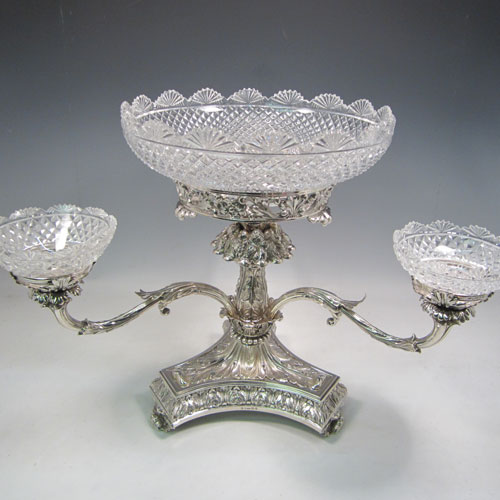The photograph showcases an intricately designed, silver-based decoration that appears both antique and elegant. Dominating the center of the image is a large, crystal-like bowl, flanked on either side by two smaller crystal bowls, each about a third the size of the central bowl. The silver base, which is vertically aligned, features elaborate and delicate detailing. The background transitions from a light gray at the bottom to a darker gray at the top, with the corners shading into black, creating subtle shadowing that accentuates the fragility and shimmer of the crystal bowls. This decorative piece, possibly intended as a serving dish or a vase, is designed to hold various items, whether solid edibles or possibly liquids, making it both functional and aesthetically pleasing.